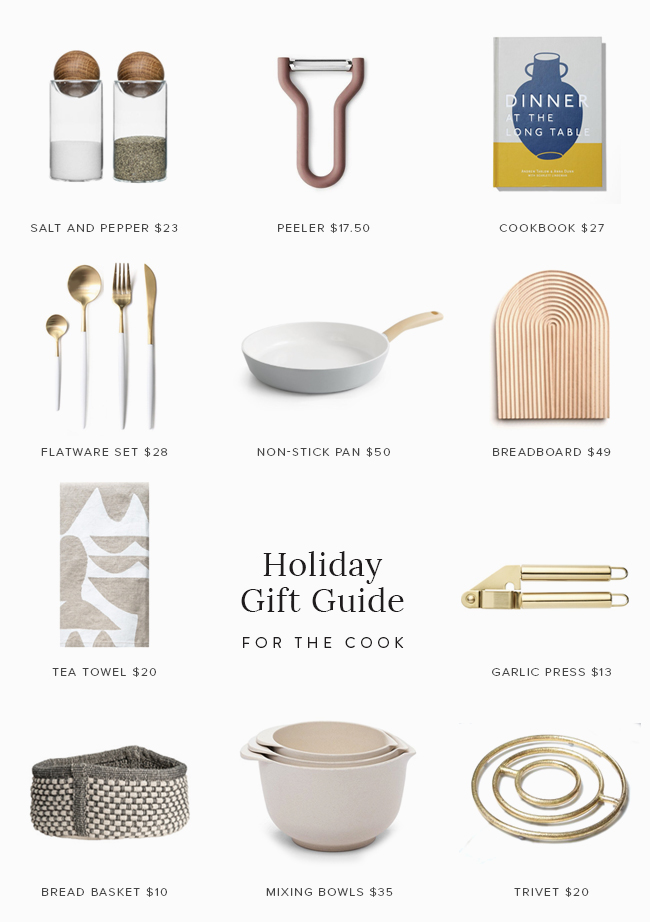This image showcases a variety of kitchen essentials against a pale gray background, each item labeled with its name and price. At the top left, there is a sleek salt and pepper shaker set priced at $23. Just to the right, a modern vegetable peeler is listed for $17.50. Below it, a beautifully illustrated cookbook is available for $27. 

A shiny flatware set, comprised of polished utensils, is marked at $28, while a pristine white nonstick pan is tagged at $50. To the right of the pan, a robust bread board, perfect for slicing and serving, is priced at $49. Nearby, a tea towel with a minimalist design is labeled $20.

Toward the bottom, the text "Holiday Gift Guide for the Cook" suggests these items as perfect presents for culinary enthusiasts. A durable garlic press is available for $13, and a classic bread basket is priced at $10. A trio of mixing bowls is shown next, costing $35 for the set. Finally, a gold-hued trivet, which combines functionality with elegance, is priced at $20. This collection is set against a soft, pale gray background, beautifully highlighting each item.